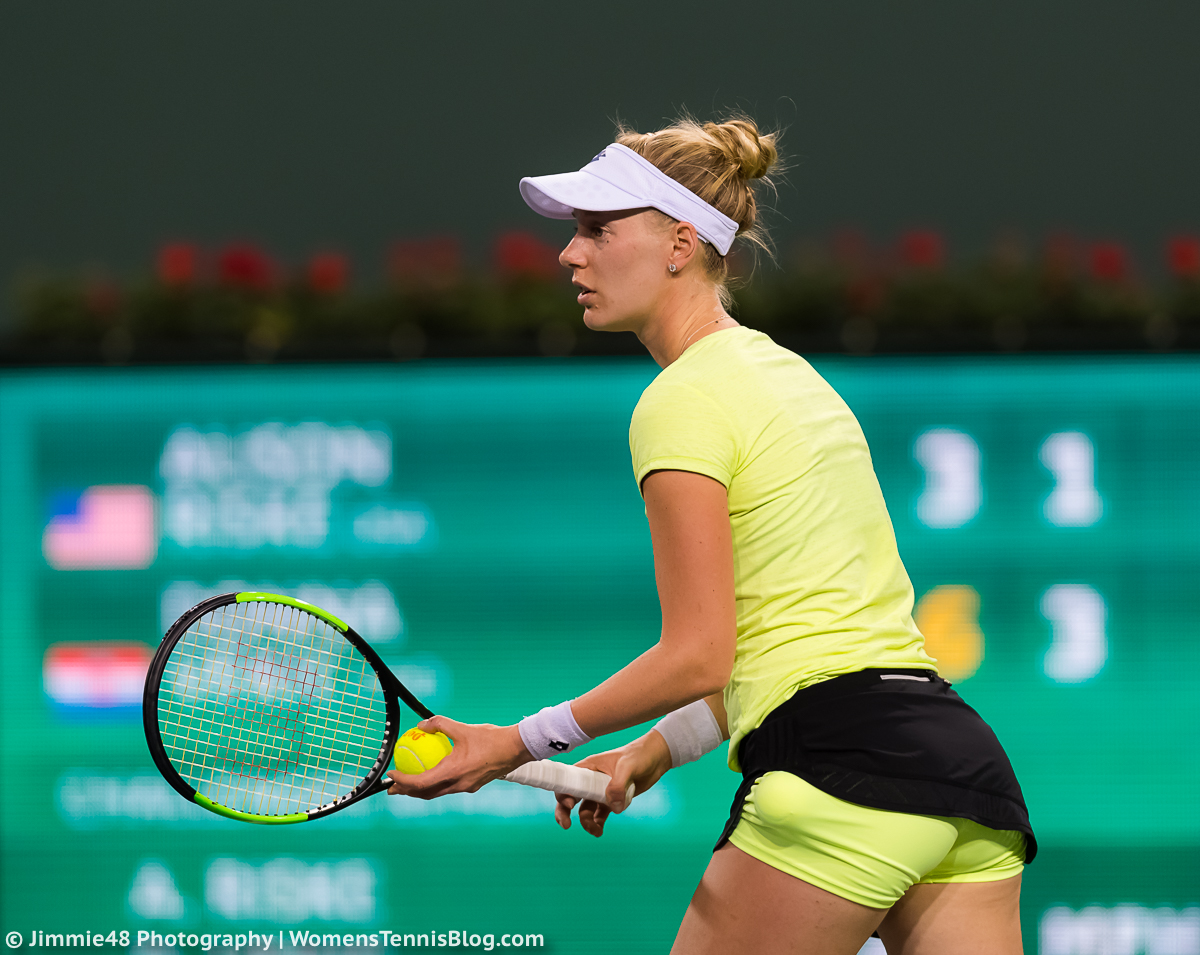The photograph captures a side profile and approximately three-quarters of a female tennis player, likely in her mid to late 20s and of Caucasian descent, actively engaged in her game. She has blonde hair pulled back into a bun, with any loose strands kept off her face by a white visor. Her outfit consists of a muted neon yellow, almost lime green short-sleeved top made of a tight, exercise-appropriate material, and matching shorts. Though she appears to be wearing a very short black tennis skirt, it's possible it has ridden up to reveal her matching yellow undershorts. A tennis ball is precariously tucked into a pocket of these shorts. On her right hand, she grips a black tennis racket accented with green and a white handle, while she holds a neon greenish yellow tennis ball in her left hand, poised as if preparing to serve. She also has wrist tape for additional support. In the background, a blurry scoreboard is visible, though unreadable. At the lower left corner, a watermark indicates the photo is credited to Jimmy 48 Photography for womenstennisblog.com.